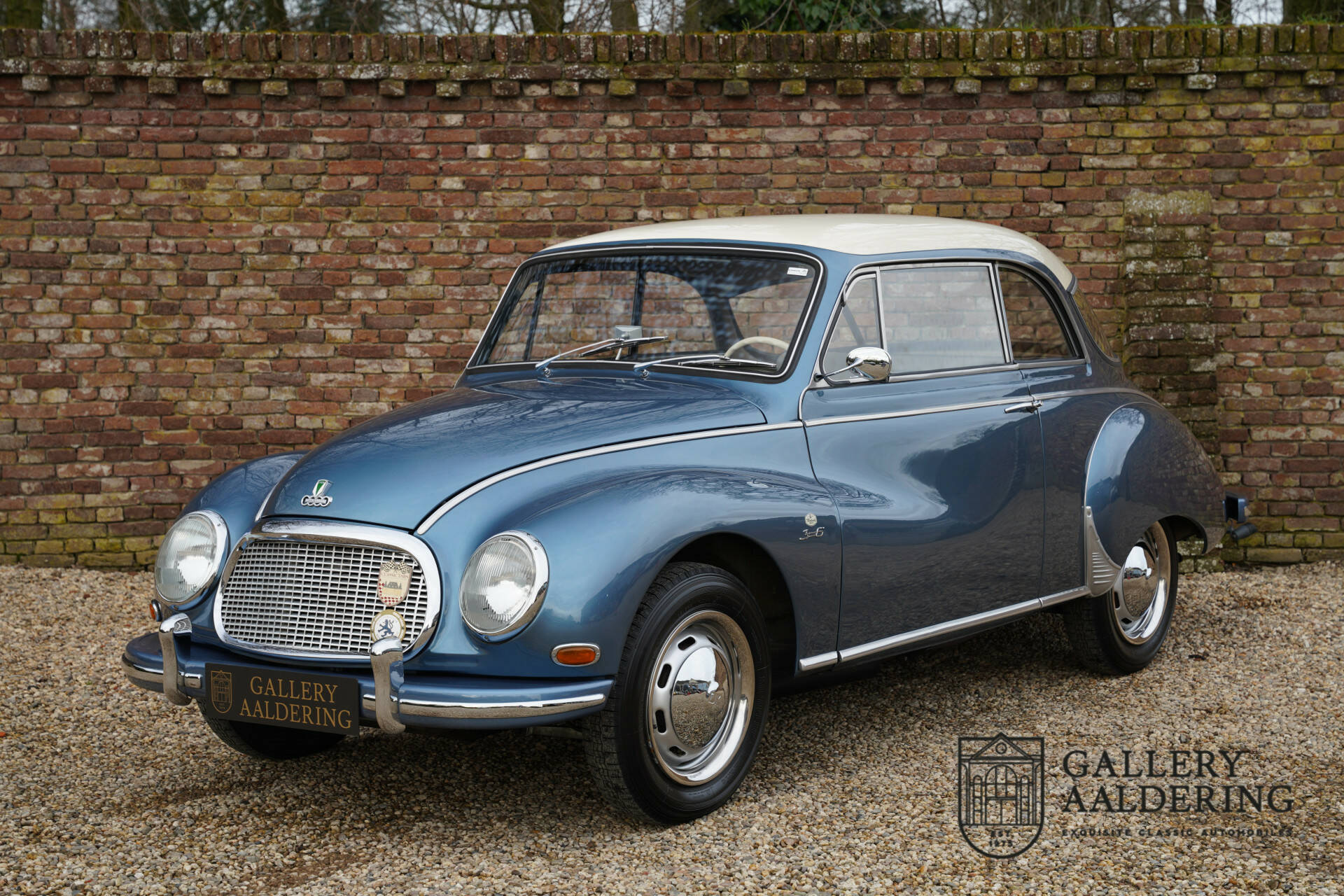The photograph showcases a meticulously restored vintage car, likely from the 1950s or early 1960s. The vehicle is an Audi, distinguished by the Audi symbol on its front hood. The car boasts a gleaming, freshly painted bluish-gray body with a contrasting white roof. Its classic design features two round headlights, two doors, and distinctive silver trim around the mirrors, windows, and chrome-plated hubcaps. The white steering wheel is visible inside the car. The front chrome bumper holds a license plate that reads "Gallery Aaldering." The car is parked at a diagonal in a gravel parking lot against a large, red and white brick wall, which shows signs of green mildew. Behind the wall, a row of trees is visible. The crisp, clean finish of the car and its impeccable condition highlight its classic charm.